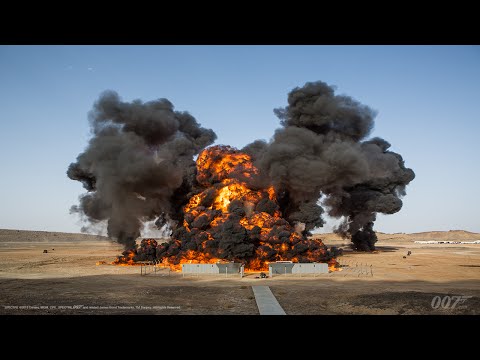This is a detailed still shot from a James Bond movie, identifiable by the 007 watermark in the bottom right corner and an additional small white text in the bottom left. The image captures a dramatic scene of an explosion in a desert or very dry area under a clear blue sky. In the center, a massive fireball erupts from a building complex, surrounded by colossal plumes of black smoke rising into the air. The complex is enclosed by a barbed wire and chain-link fence, with some concrete walls visible near the front. Leading to the structure, there's a concrete sidewalk bordered by extensive stretches of dark brown dirt or sandy ground. The explosion dominates the middle of the image, while far in the distance, another building complex can be seen. The foreground and immediate surroundings suggest a barren environment, with dead or yellowed grass visible. The top and bottom sections of the image feature thin rectangular black areas, framing the explosive action that takes center stage.